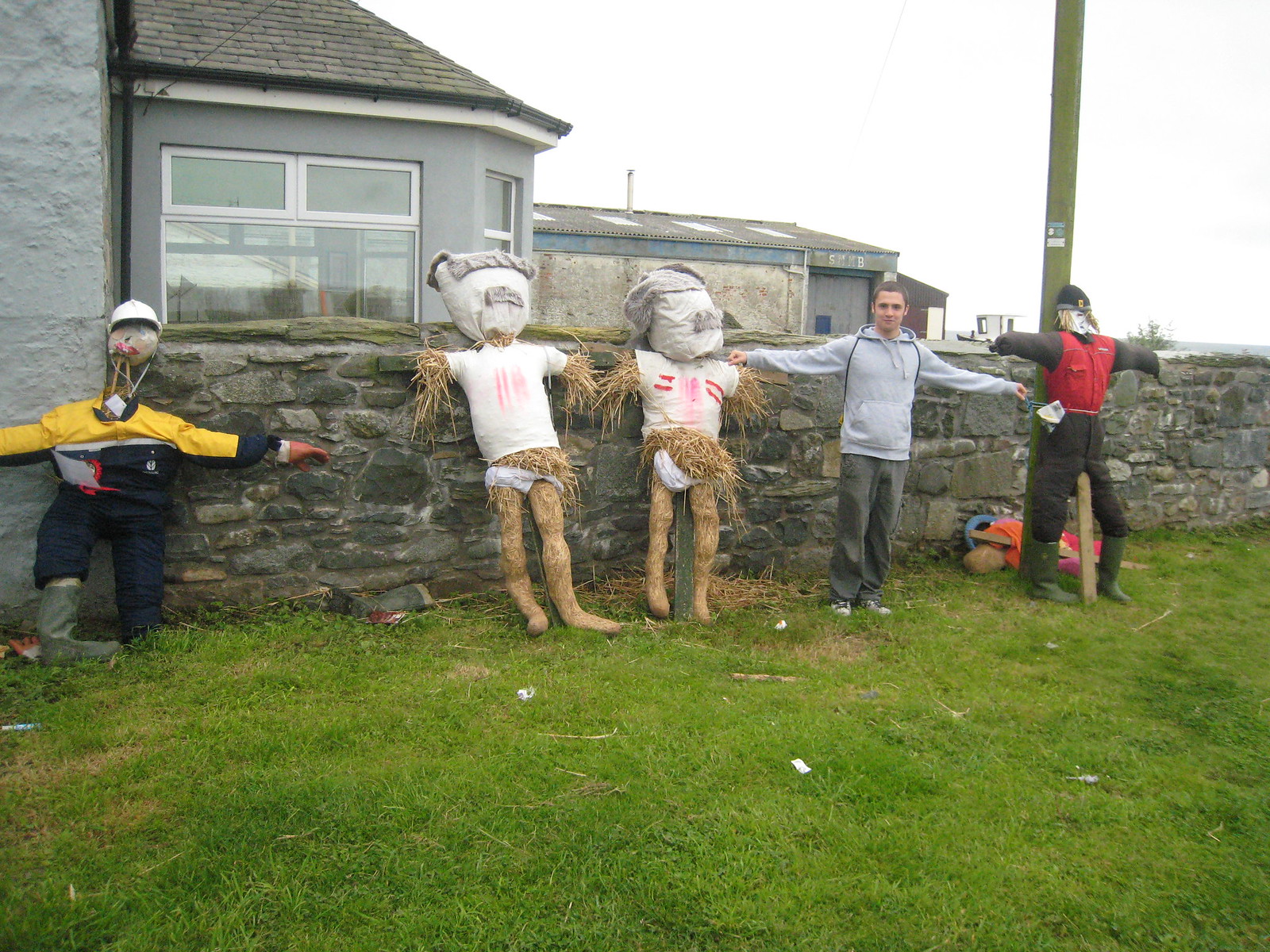A daylight, outdoor photograph captures a whimsical scene in the yard of an Irish-style home with a gray stone facade. Dominating the foreground is a fairly high stone and gravel wall, running horizontally from the left side of the image to the right. Behind this wall, the gray stone building features a prominent bay window, and in the distance, another structure appears to be a farm building or large garage, set against a white, smoky sky in the top right corner.

Leaning against this stone wall are four scarecrows and one human figure, all positioned to create a visual tableau. The real person, approximately 16 years old, is standing left of center, dressed in a gray tank top with a hoodie and dark gray pants, mimicking the stance of the scarecrows. On the far left stands a shorter scarecrow dressed in a yellow jacket and black pants. Next to the human on his left are two scarecrows with white pillowcase heads stuffed with straw, each clad in white shirts and what appear to be white tighty-whitie underwear, with straw spilling out from various openings, giving them an almost comically disheveled appearance. Their makeshift 'hair' is fashioned from different pieces of clothing on top of the pillowcases. To the right of the human figure is another scarecrow, attached to a utility pole, wearing a red vest, a black shirt, black pants, and a ball cap, completing the scene.

The backdrop of the photograph, characterized by an overcast sky, further enhances the quirky assembly of scarecrows and the young boy, all standing on a carpet of green grass. No text or other markings are present in the image, allowing the curious arrangement of scarecrows and the authentic architecture to take center stage.